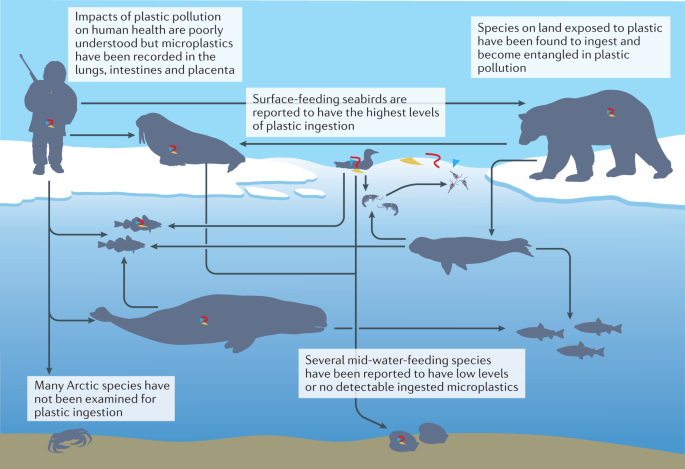The image is a detailed, computer-generated illustration commonly found in educational textbooks. It depicts the impacts of plastic pollution on various Arctic species through a clear and informative visual representation. The background transitions from lighter blue at the surface to darker blue as it goes deeper, concluding with a brown sandy seabed. 

Above the water, there is an ice-covered landmass with silhouettes of an Eskimo man, a polar bear, and a walrus. White arrows point to these animals, accompanied by text boxes explaining how plastic pollution affects terrestrial and marine life. One text box states, "Species on land exposed to plastic have been found to ingest and become entangled in plastic pollution."

In the ocean foreground, a seabird floats on the water's surface. Another arrow indicates that "Surface-feeding seabirds are reported to have the highest levels of plastic ingestion." Various sea creatures, including fish, seals, dolphins, crabs, and shellfish, are depicted at different depths in the water and on the seabed. Notably, one section of the text highlights that "Many Arctic species have not been examined for plastic ingestion," while another indicates that "Several mid-water feeding species have been reported to have low levels or no detectable ingested microplastics."

The diagram is labeled with a significant note: "Impacts of plastic pollution on human health are poorly understood, but microplastics have been recorded in the lungs, intestines, and placenta." This comprehensive visual serves as an informative resource on the pervasive issue of plastic pollution and its largely unknown consequences on wildlife and human health.